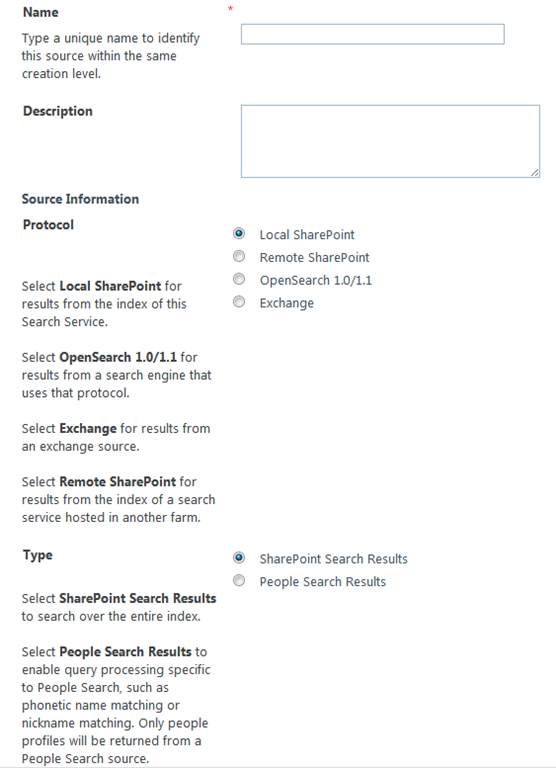The image showcases a minimalist form with a white background and black text, designed for configuring search sources. The form contains various input fields and buttons arranged horizontally and vertically. 

At the top, a text box is labeled "Name," with an instruction to enter a unique identifier for the source within the same creation level. 

Below, a "Description" text area is available for additional information.

The form then dives into protocol settings with a detailed explanation:
- **Local SharePoint:** Preselected, it retrieves results from the index of the current search service.
- **OpenSearch 1.0/1.1:** Fetches results from search engines using this protocol.
- **Exchange:** Acquires results from an Exchange source.
- **Remote SharePoint:** Gathers results from the index of a search service hosted in a different farm.

Next, the form presents type options for search results:
- **SharePoint Search Results:** Preselected, allowing a broad search over the entire index.
- **People Search Results:** Specifically enables query processing tailored to people searches, including phonetic and nickname matching, returning only profiles relevant to the search.

This form, though simple in design, is detailed and functional, providing users with clear steps and options for configuring their search sources efficiently.